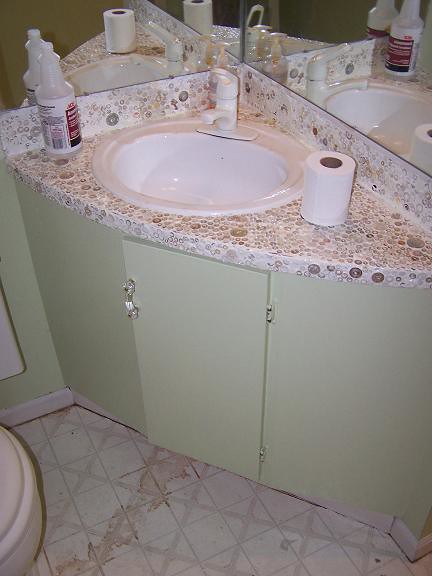The photo captures a detailed view of a bathroom corner from an angled, downward perspective. Dominating the center of the image is a white bathroom sink, accompanied by a matching white water spout and hand nozzle. The sink is set into a countertop that surrounds it, designed with a white base embellished with a brown, circular floral pattern. 

To the immediate right of the sink on the countertop, there is a half-used roll of toilet paper. On the left side of the sink, a clear bottle with a white and red label—likely a bathroom cleaner—stands prominently. Behind the spout of the sink sits a container of gold-colored hand soap, adding a touch of elegance to the setting. 

This corner placement brings two glass mirrors into view, converging where the walls meet and reflecting the elements of the bathroom. Below the sink, olive green painted wallpaper and an olive green cupboard with a central door and several hinges provide a soothing contrast to the predominantly white hues. 

The flooring is made up of white tiles with gray outlines, enhancing the brightness of the space. A small portion of a toilet is visible at the bottom left corner of the photo, hinting at the layout of the rest of the bathroom beyond the frame.